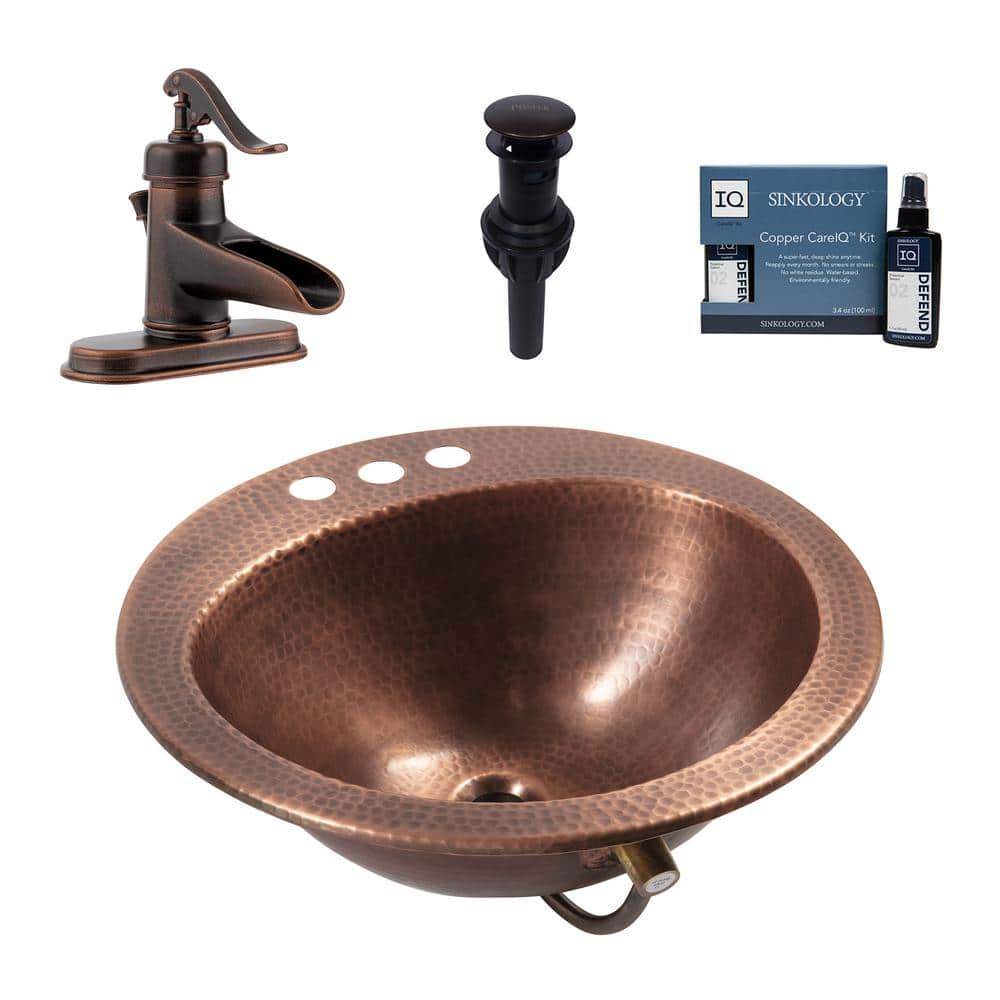This image features a beautifully crafted round copper sink, prominently displayed in the center. The sink, which is textured with small black dots resembling a hammered brass style, lacks an attached faucet but has three pre-drilled holes at the top for faucet installation. Surrounding the sink are three distinct accessories set against a white backdrop. On the left is a vintage-style copper faucet with a cylindrical spout and an old-school lever for water control. In the middle is a black drain stopper that fits into the sink’s central hole. To the right, there is a blue box labeled "Sinkology Copper Care IQ Kit," accompanied by a black spray bottle, designed to maintain the copper's shiny, untarnished appearance. Together, these elements create an appealing and functional display, ideal for a product listing on a website.